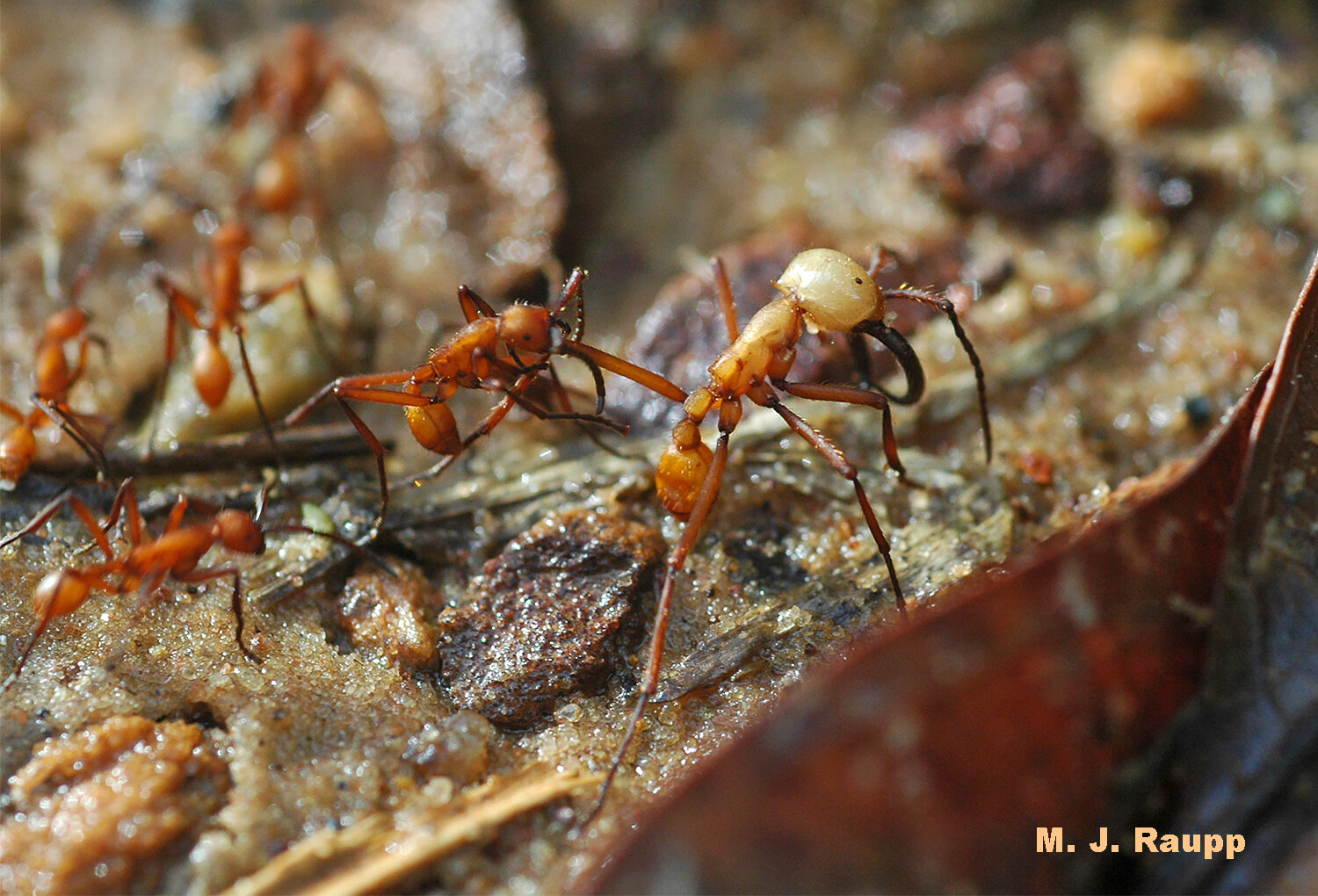The image captures a close-up view of a group of ants on a textured, brownish surface, possibly resembling raisin bread or a substance like brown sugar. Dominated by earthy hues, the photograph highlights a central, larger ant with a pale light brown body and dark pincers, its head oriented downward as if foraging. Surrounding this prominent ant are four smaller ants, also with their heads down, appearing to gather from the glittery, possibly food-like surface. The backdrop, blurred towards the top, enhances the focus on the ants' activities in the foreground. A brown leaf or piece of wood is visible in the bottom right corner, next to the photographer’s signature, "MJ Raupp (R-A-U-P-P)," etched clearly into the image.